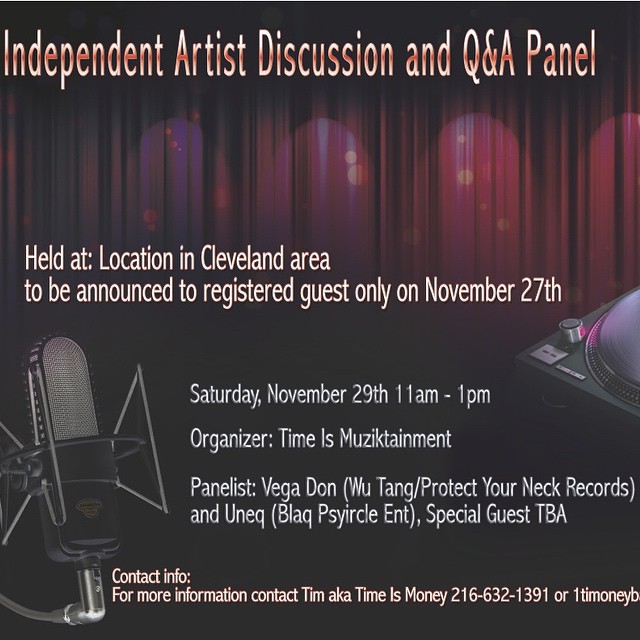This is a detailed square-shaped poster advertising an Independent Artist Discussion and Q&A Panel event. The title at the top, written in white and red, reads "Independent Artist Discussion and Q&A Panel." Directly below, the text in white states that the event will be held at a Cleveland area location to be announced to registered guests only on November 27th. The event date is further clarified in light gray text below as Saturday, November 29th from 11 a.m. to 1 p.m. The organizer, Time is Music Tainment, lists panelists including Vega Dawn from Wu-Tang's Protect Your Neck Records and Yu-Neck from Spiracle. A special guest is yet to be announced. At the bottom, in yellow text, contact information is provided: For more information, contact Tim, aka TimeIsMoney, at 216-632-1391 or via email at 1 Time Money B. The poster features a background with red curtains at the top, an old-style microphone on the bottom left, and a partially visible musical instrument on the right, all set against a black backdrop.